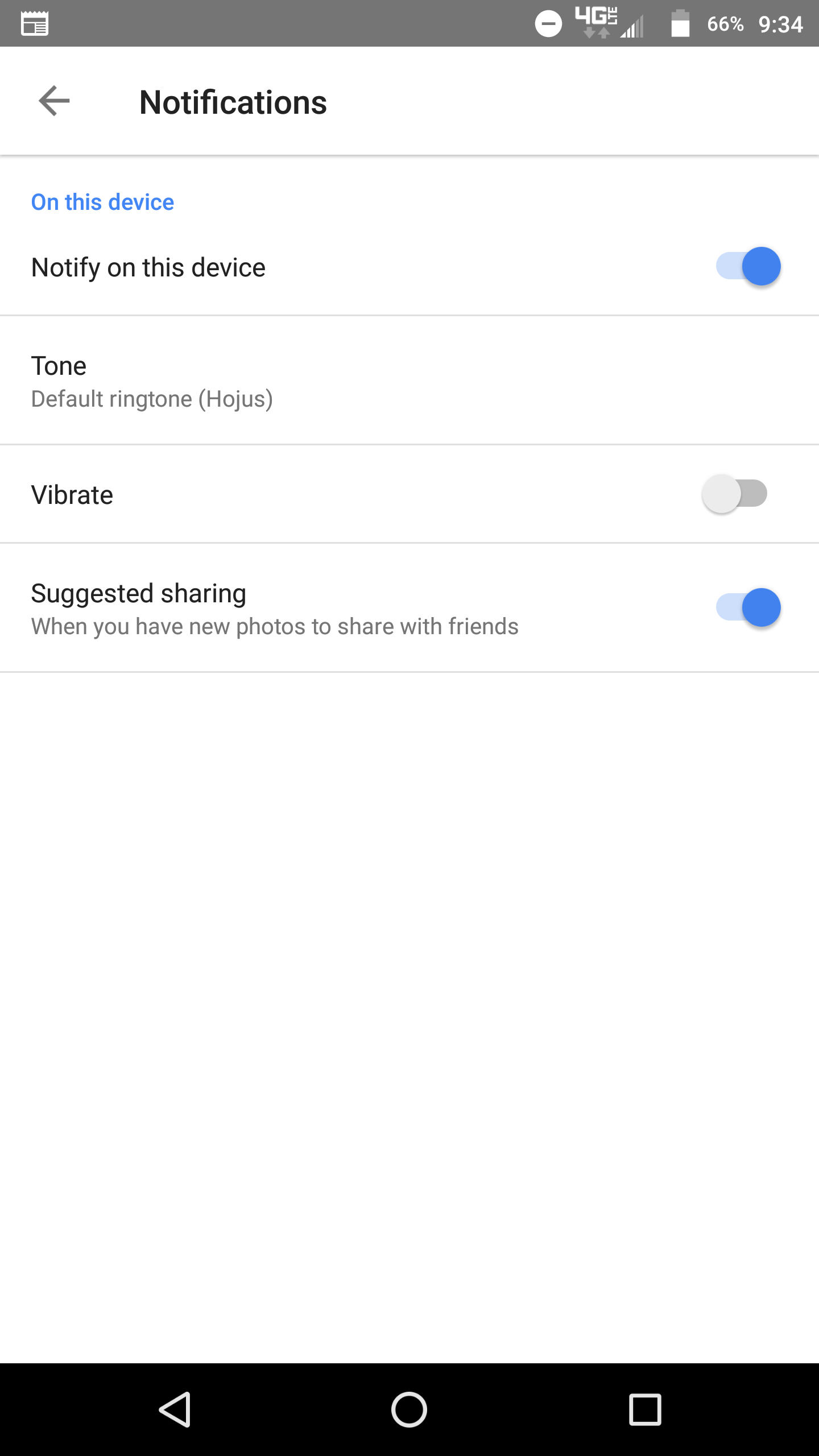The image appears to be a screenshot from a smartphone. At the top of the screen, there is a gray status bar displaying key information. On the right side, it shows a battery percentage of 66%, with an indicator that the device is connected to a 4G network. The time displayed is 9:34 AM. Moving below, the main content area has a white background.

At the top of this area, a header labeled "Notifications" is prominently displayed. The next section is demarcated by two dividers and includes a blue-highlighted label: "On this device," followed by a description: "Notify on this device." To the right of this text is a blue toggle switch, which is currently in the 'on' position.

Moving down, the next section is labeled "Tone," with the text "Default Ringtone" and the word "HOJUS" in parentheses. Below this, there is a "Vibrate" section featuring an on/off toggle button. The toggle is currently in the 'off' position, as indicated by its grey color.

The following section is titled "Suggested Sharing," with an explanatory note stating: "When you have new photos to share with friends." To the right of this note, there is another toggle switch, which is turned on and highlighted in blue.

Beneath these sections, there is a blank white space, leading to a black border at the bottom of the screen. This black border contains three icons commonly found in smartphone navigation bars: a left-pointing triangle, a circle in the middle, and a square on the right side.

The overall layout suggests a settings menu related to notifications and sharing preferences.